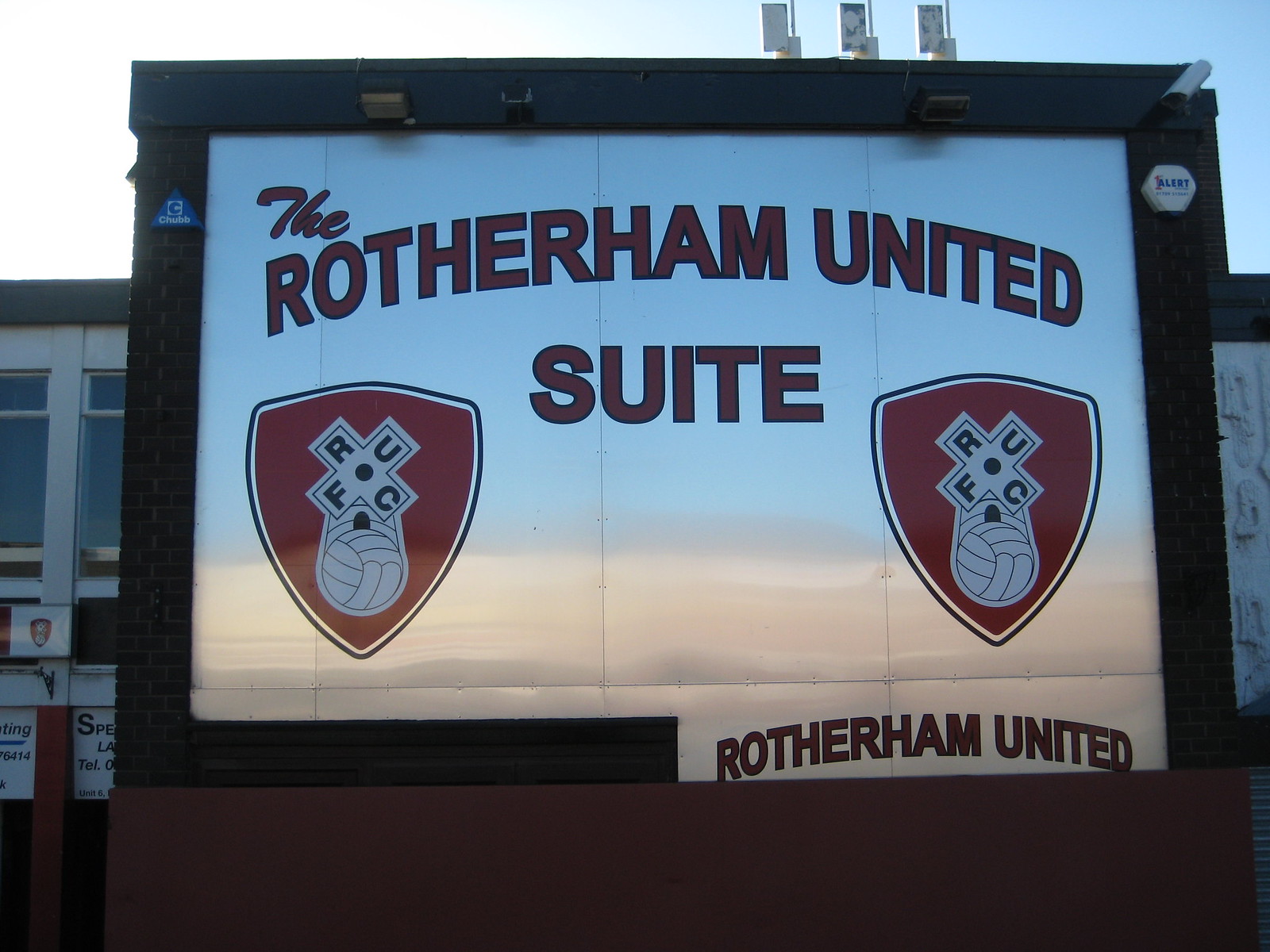The sign, prominently bordered by a black, wooden-like frame, lies in the center, featuring a white background with detailed text and crests. Above the frame, there's a camera positioned in the top right corner and two spotlights that provide illumination from the top. The sign, likely made of metal, reads "The Rotherham United Suite" in bold red text with a black outline in the upper portion, while the bottom right corner states "Rotherham United." Flanking the text are two identical crests positioned at the bottom left and right. Each crest consists of a shield with a soccer ball in the middle forming a windmill-like design and bears the acronym "RUFC." Behind the sign, a building with windows is visible, and the background showcases a clear blue sky.